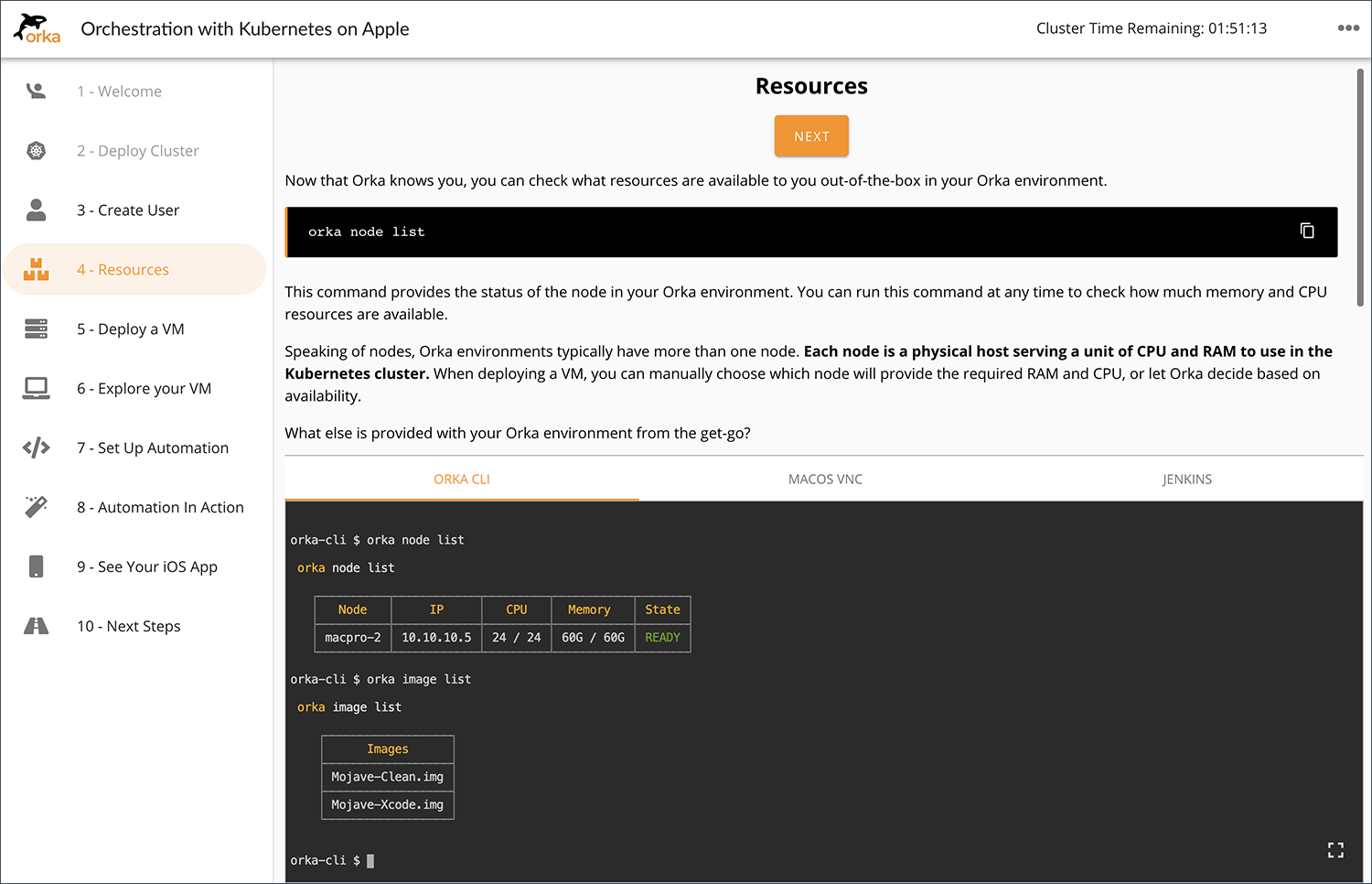### Detailed Caption for the Screen Capture of the Website

This screen capture depicts a section of a website with a primary focus on Kubernetes orchestration through a service called "Orange Orca". At the top of the image, there's a distinct white strip featuring a black whale icon, adjacent to the title "Orange Orca" in orange font. Below the title, a subheading in black font reads "Orchestration with Kubernetes," followed by a status indicator displaying "Cluster time remaining: 1 hour, 51 minutes, and 13 seconds." Beside this status, three gray ellipsis dots are positioned.

On the left-hand side of the screen, a side menu panel is presented against a white background. The menu items, listed in gray font, include various options such as:

- **Welcome** with an abstract waving person icon.
- **Deploy Cluster** symbolized with a circular icon.
- **Create User** illustrated by a head-and-shoulders icon.
- **Resources** represented by a stack of books; this option is highlighted in a light orange box with dark orange font.

Additional menu items continue further below:
- **Deploy a VM** with a boxes icon.
- **Explore your VM** featuring a computer icon.
- **Set Up Automation** illustrated by two triangular shapes.
- **Automation in Action** marked with a magic wand icon.
- **See Your iOS App** showcasing a cellphone icon.
- **Next Steps** depicted with a road icon.

The central portion of the image focuses on resource information. A black title reads "Resources", followed by an orange highlighted note, "Know that Orca knows you." The description elaborates that users can view the resources available to them in their Orca environment out-of-the-box.

Center screen, a black box labeled "Orca Node List" contains text explaining that this command can be used any time to check the status, memory, and CPU resources of nodes within the environment. The explanation provided emphasizes the typical multi-node structure of Orca environments, outlining how each node serves as a physical host that provides CPU and RAM resources to the Kubernetes cluster. It also details options for deploying a VM, including manually choosing a node or letting Orca automatically select based on resource availability.

Further down, a gray box titled "Orca CLI" mentions features like "Make," "Host VNC," and "Jenkins." Within this section, the user can see a mixture of white, orange, and green text and various numbers, indicating command lines or code snippets. Closing the capture, a white square is visible at the very bottom.